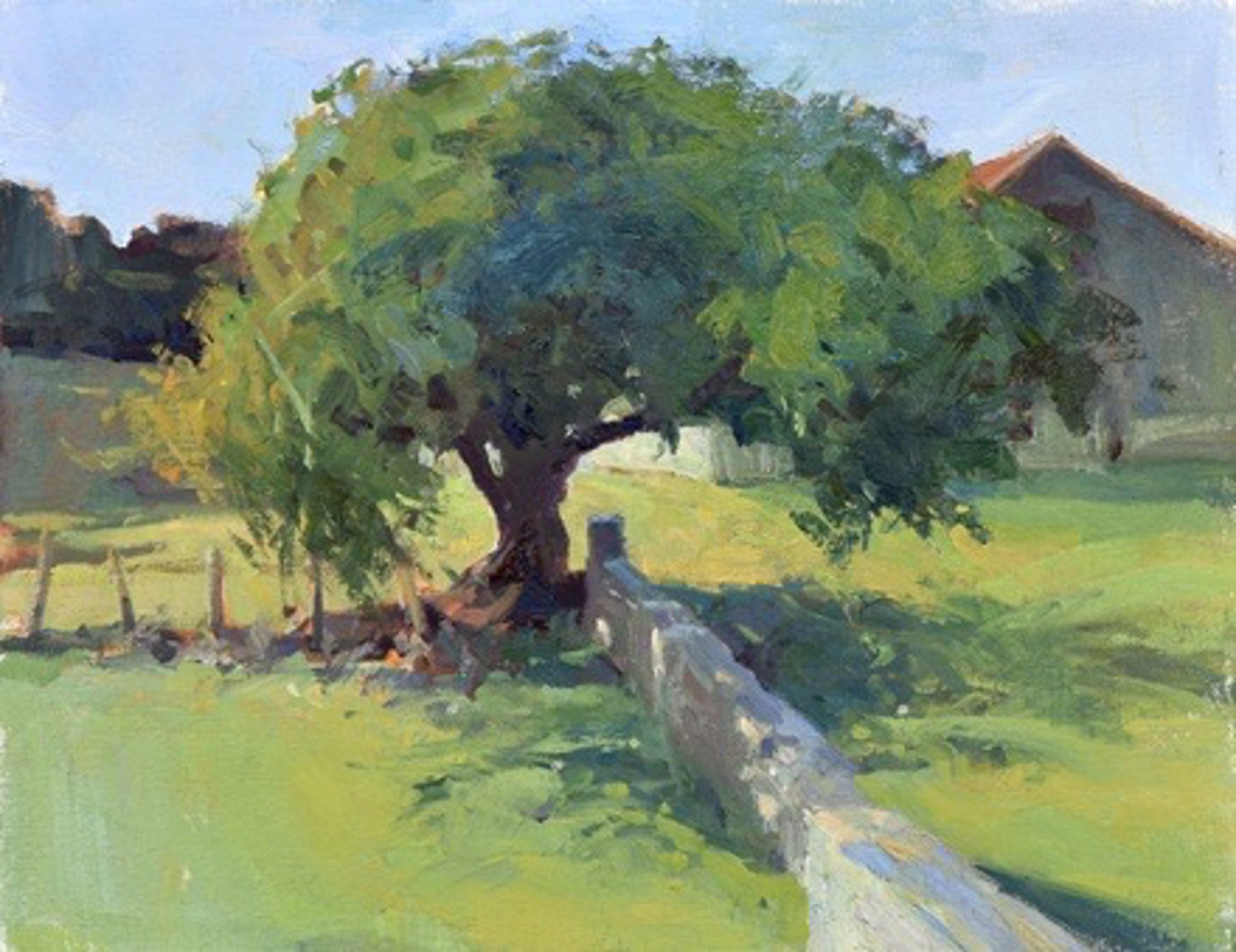The image depicts an impressionist-style watercolor painting of a vibrant rural scene. The central focus is a large tree with a wide trunk and an expansive canopy, casting reddish shadows over the lush green grass. To the left of the tree, a little stone wall stretches for about 20 feet, ending near the tree, and a wooden fence extends from the tree to the left. In the right background, partially obscured by branches, is a barn or farmhouse with a red or orange roof and white siding. The blue sky is clear, stretching across the scene, complementing the green grass below. The painting captures additional elements like brown mountains in the distance, contributing to the peaceful, pleasant farmland atmosphere. The artwork utilizes broad strokes of color to create texture and depth, resulting in a deceptively simple, yet clear and proportionate image.